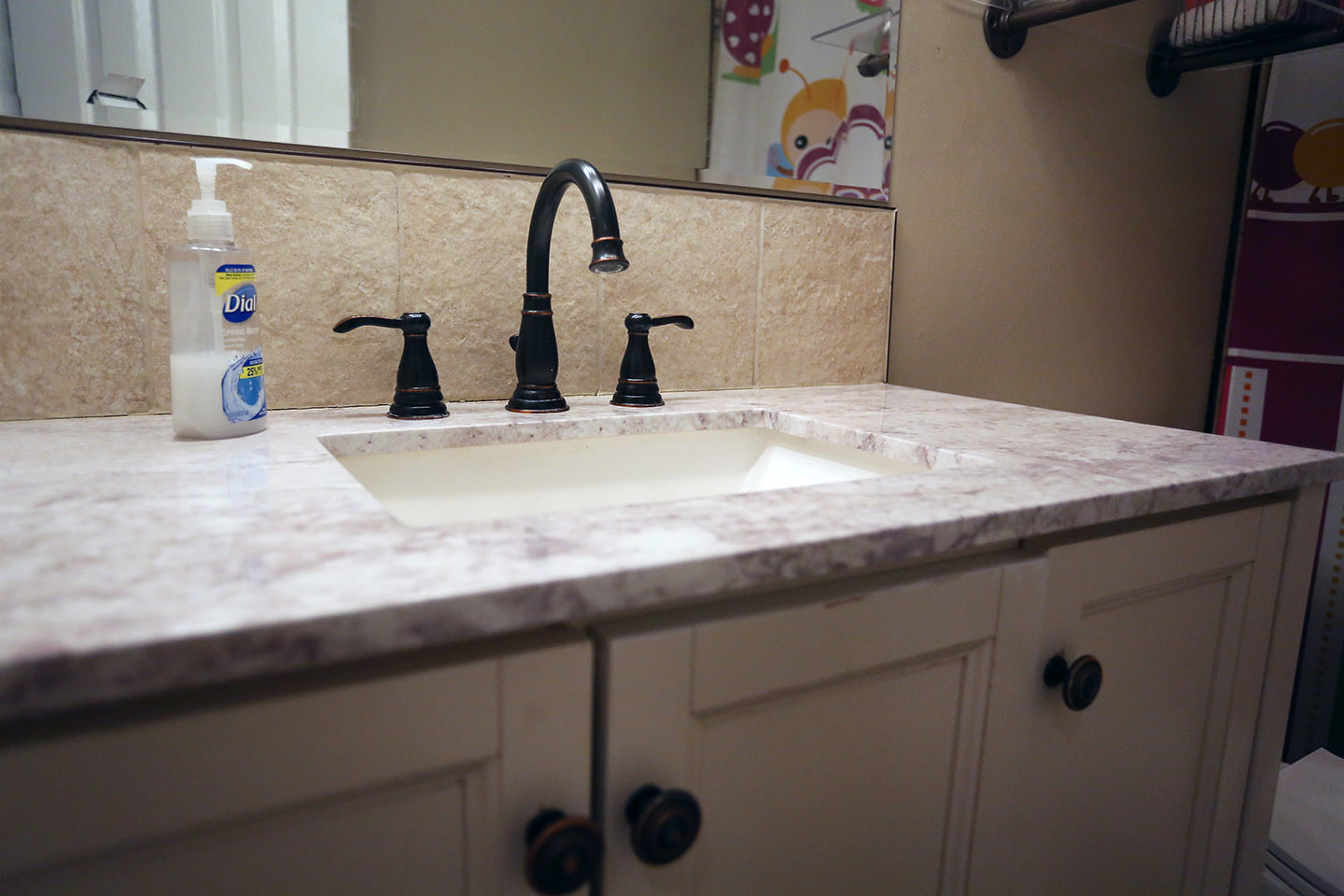A detailed view of a bathroom is captured, showcasing a sink area composed of a marbled countertop in a blend of white and reddish-brown hues. Beneath the sink, there are cabinets adorned with round knobs. To the right of the sink, mounted hooks are available for hanging bath towels. The mirror above the sink reflects part of the shower curtain to its right and the white doorway of the bathroom to its left, adding depth to the scene.